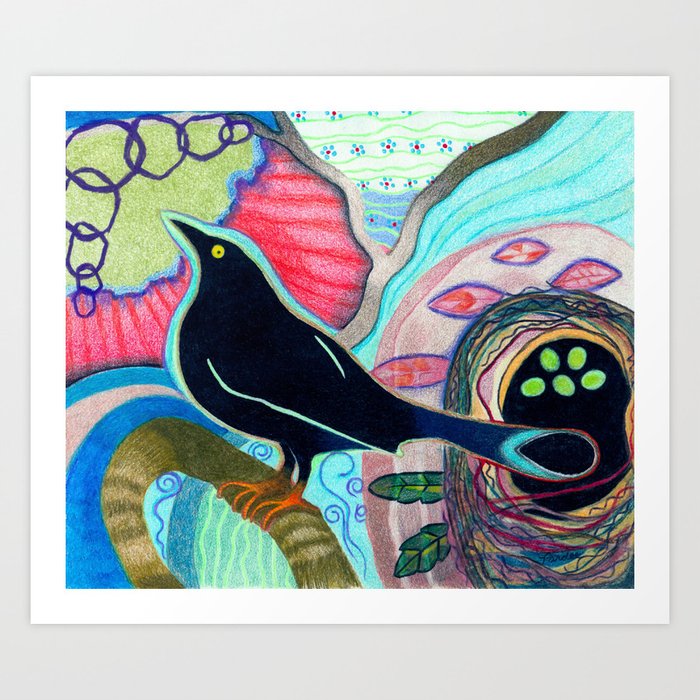The image is a colorful, childlike crayon painting set against a gray background with a white border. It depicts a black crow with an intricate blue aura surrounding its beak, stomach, and upper body, extending partially to its tail, which also transitions into pink hues. The crow stands with orange feet on a warped branch made of brown and light yellow, with patches of blue and white stripes. The background is a chaotic blend of vibrant patterns and shapes—circles of various colors including purple, red, green, and white; swirls and curved rings; and randomly placed lines. To the bottom right of the painting, a nest appears with five green, oblong objects resembling eggs. The nest is encircled by blue lines and shapes. At the top left, a red, yellow, purple, and blue circular shape with internal circles can be seen. The overall composition exudes a playful, almost surreal quality filled with whimsical details.